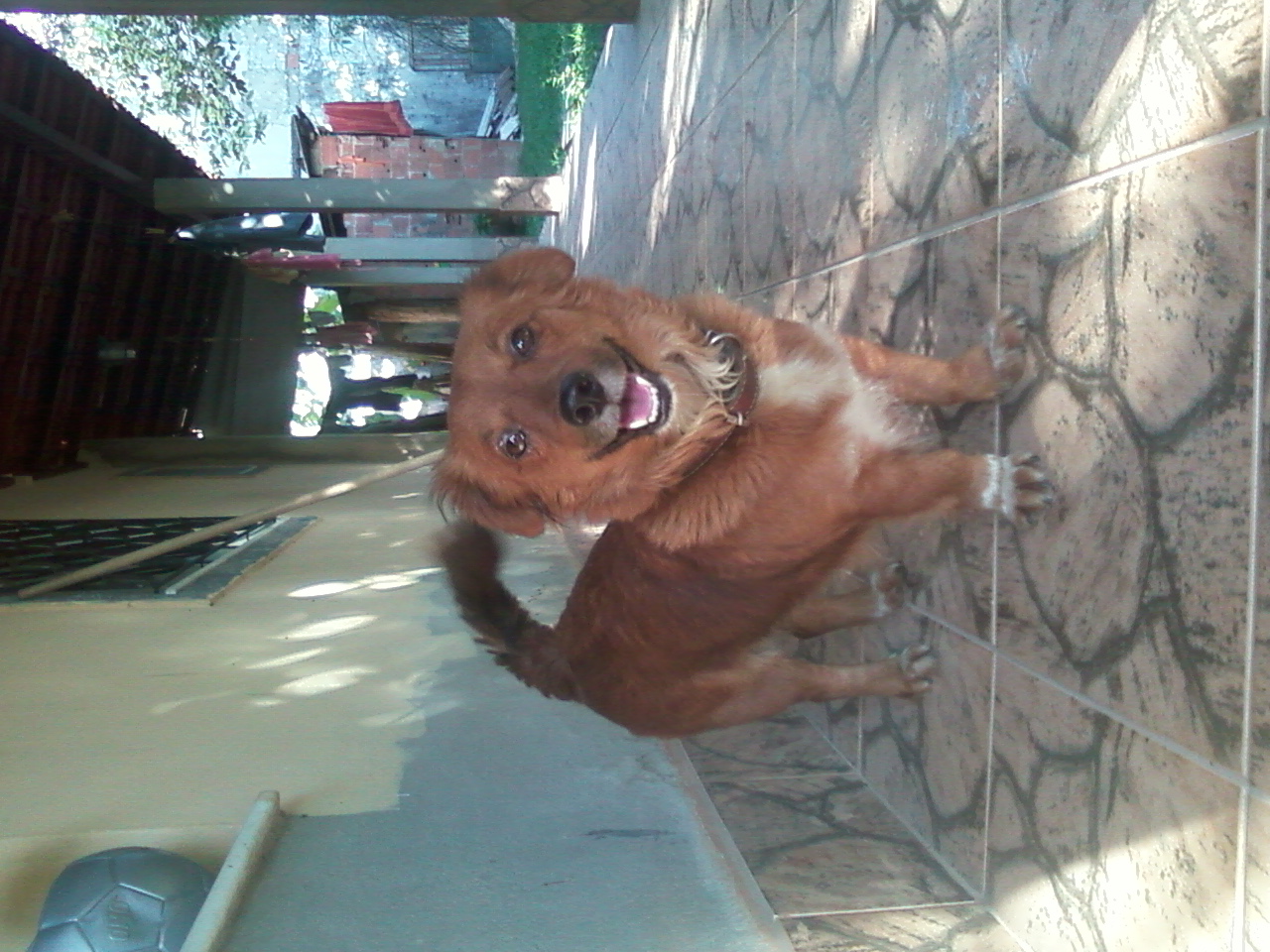This rectangular photograph, taken outdoors and turned sideways, features a young, small mixed-breed dog with a medium-length coat. The dog is predominantly brown with a touch of black on its curved tail, white fur on its chest and feet, and light tan markings. A brown leather collar with a silver ring adorns the dog's neck. The dog stands on a smooth, tiled patio made of large, brown square tiles. Behind the dog is a partially painted building wall, the lower section covered in silvery blue paint while the upper part remains a yellow cream color. A window with metal security bars is set into the wall. The patio has a roof extending overhead, offering some shade. To the right, bright sunlight illuminates a grassy area with green trees. Concrete pillars align along the wall and patio, leading to a small brick structure in the background.